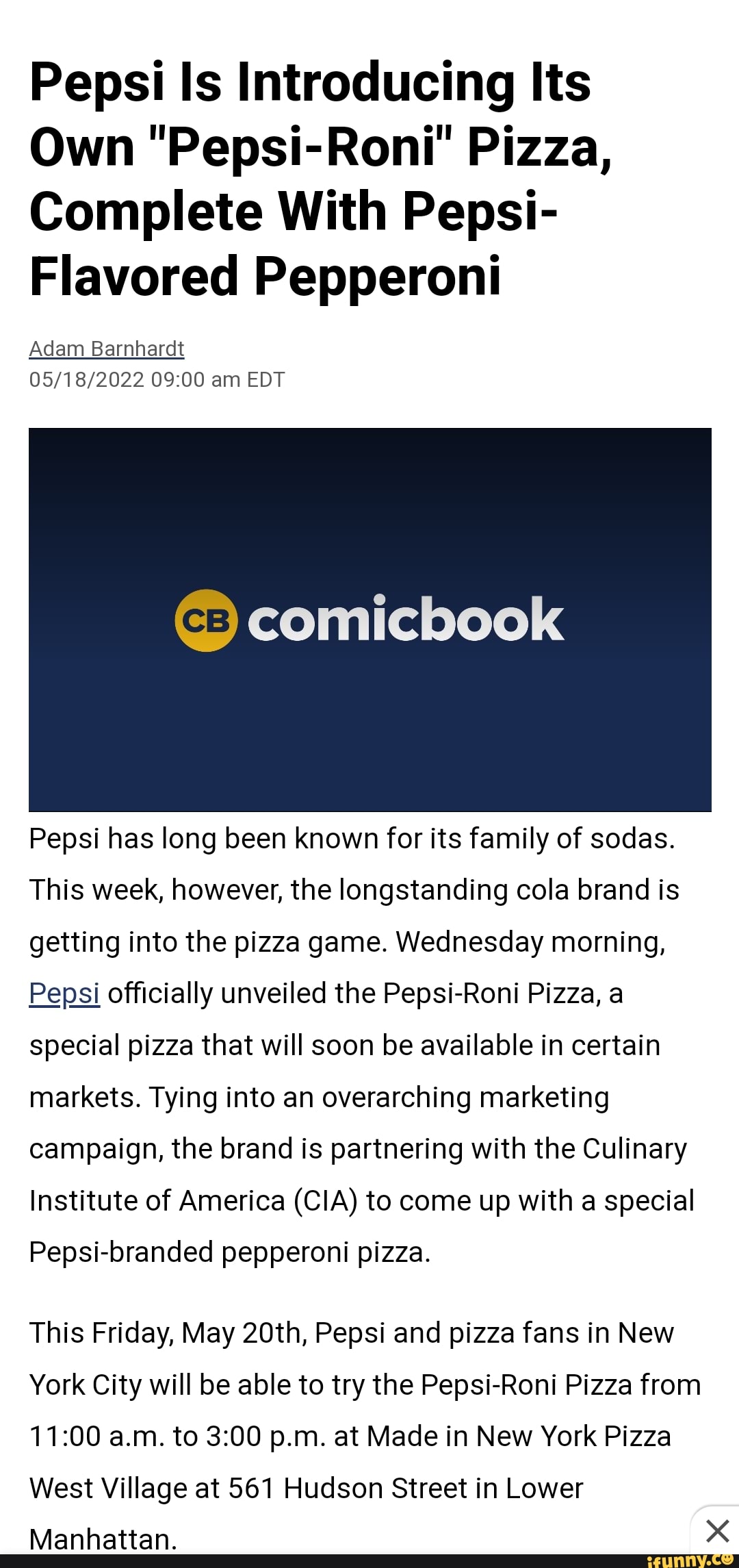Here's a cleaned-up and detailed caption:

---

The image, captured from a phone screen, details an article by Adam Barnhart dated May 18, 2022, at 9:00 a.m. EDT, hosted on the ComicBook.com website, identifiable by the navy rectangle with the word "ComicBook" and a yellow "CB" emblem at the top. The article announces Pepsi’s introduction of the "Pepsi Roni" pizza, featuring Pepsi-flavored pepperoni. This innovative product is part of Pepsi's foray into the pizza market, achieved in collaboration with the Culinary Institute of America (CIA). The specialty pizza will be available for tasting in New York City on Friday, May 20th, from 11 a.m. to 3 p.m. at Made in New York Pizza located at 561 Hudson Street in the West Village, Lower Manhattan.